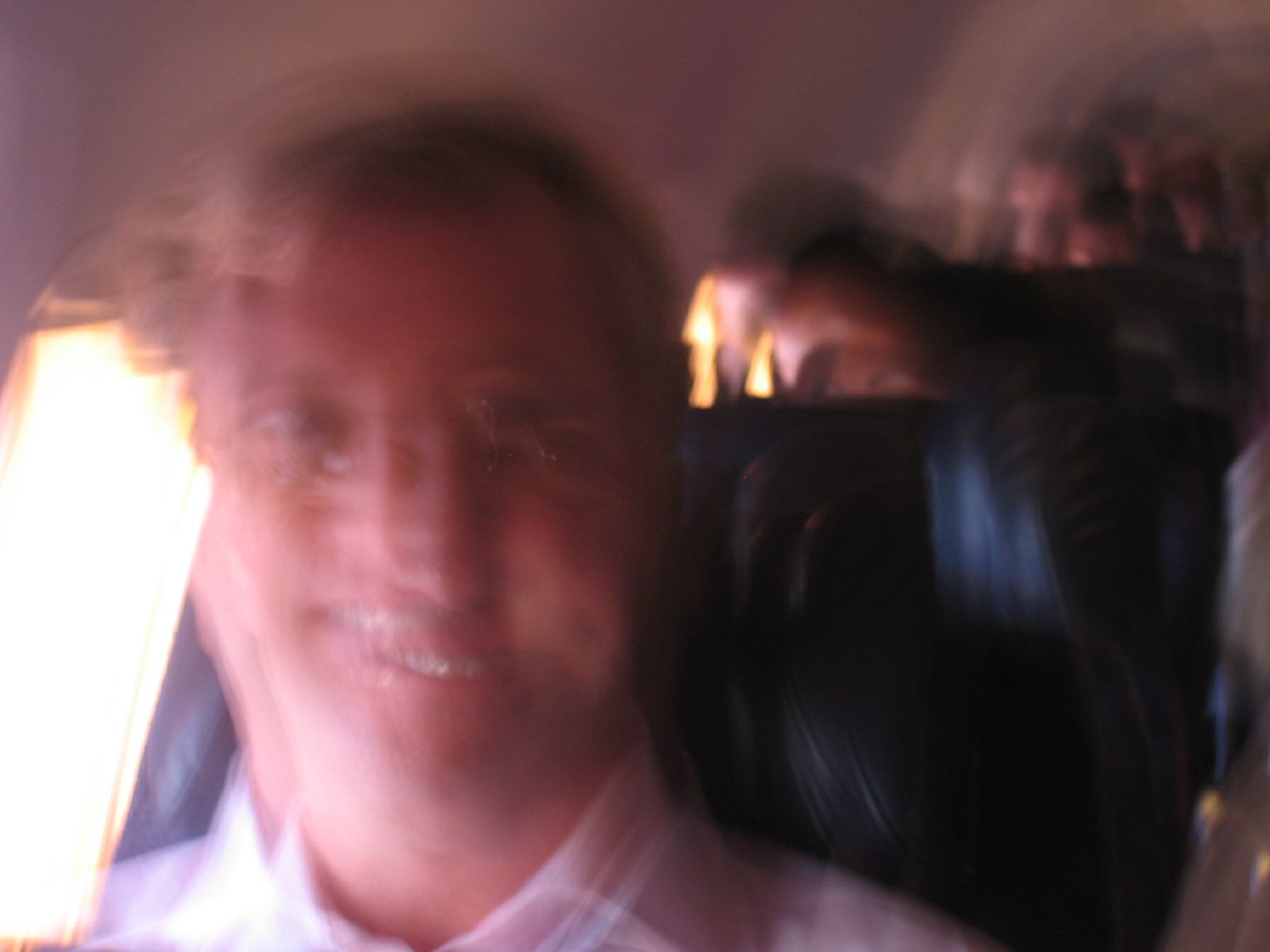The image depicts an extremely blurry interior of a plane, resembling a time-lapse or motion blur effect, where details seem layered or duplicated. At the forefront is a white middle-aged man with short gray hair, smiling with his mouth open, exposing his teeth. His facial features appear duplicated due to the blurriness, giving him a phantasmic appearance. He is wearing a collared, possibly plaid, shirt and sits by a window with light streaming through. The windows are square-shaped, and the man sits in a blue or possibly black leather-padded seat. The plane's cabin features white walls and several indistinct human figures in the background, also affected by the blur, seated in blue chairs.